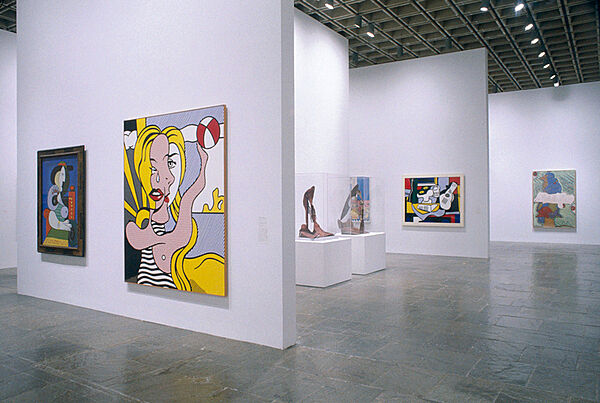The photograph captures the interior of a modern art gallery featuring an array of detailed elements. The gallery’s white drywall forms a U-shaped layout that directs the viewer's eye throughout the room. The reflective marble or stone-tiled floor is arranged in a square pattern, contributing to the room’s sleek aesthetic. The ceiling is composed of a black grid with multiple drop lights illuminating the artwork below. Along the white walls, various abstract paintings are displayed, including a prominent portrait of a woman with blonde hair and red lipstick on the left side. This piece is next to another painting framed in brown, showcasing a dual-faced character against a blue background, surrounded by a palette of red, blue, white, and orange. Central to the room, two cube-shaped pedestals with glass coverings display brass sculptures. On the outer left-hand wall, two notable artworks catch the eye: one, a woman in a black-and-white striped swimsuit against a beach-like backdrop, rendered with multiple facial perspectives; the other, a cartoonish figure standing to the right against a blue background, framed in black and featuring a blend of gray, blue, green, red, white, and black colors. The gallery’s minimalist and well-lit environment highlights the abstract and interpretive nature of the displayed art, encouraging detailed observation and interpretation.